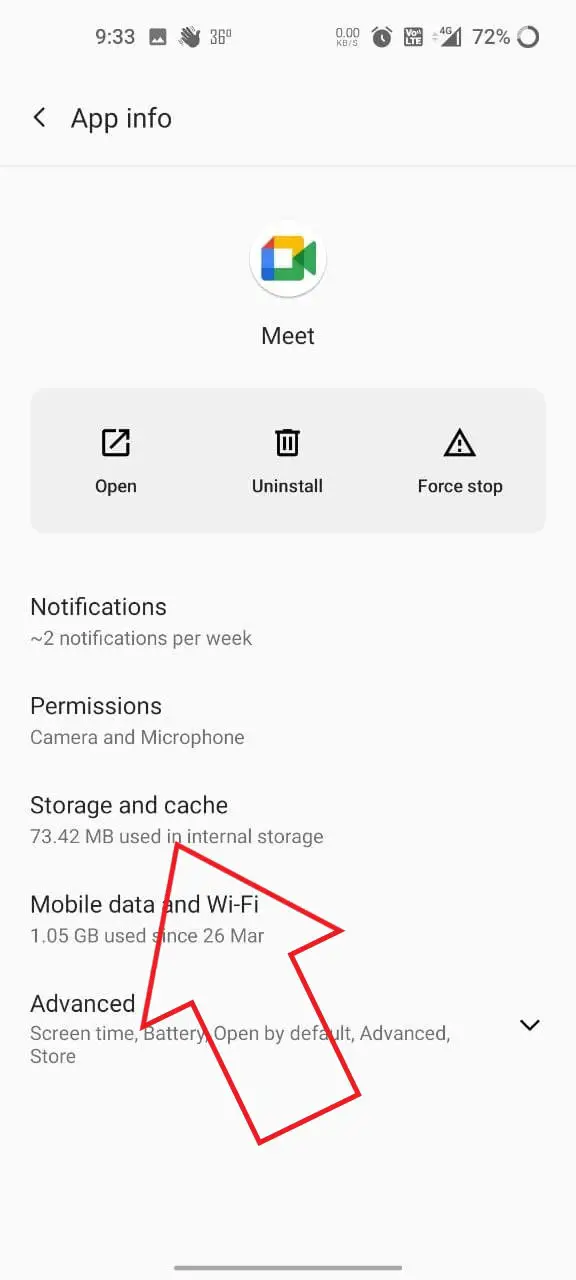This is a detailed and descriptive caption for the provided image:

The image is a screenshot taken from a cell phone. At the top of the screen, the time displayed is 9:33. Several icons are present there, including a battery indicator that is depicted as a circular graphic. The circle is filled to 72%, with the filled section in dark gray and the remaining 28% in light gray, representing the battery level.

In the upper middle section of the screenshot is an icon of a video camera in Google colors, labeled "Meet" underneath. Below this, a rectangular menu with three options is shown. From left to right, the options are "Open," "Uninstall" (with an icon resembling a trash can), and "Force Stop" (with a warning triangle containing an exclamation point inside).

On the left side of the screen, a list of options is visible, which includes "Notifications," "Permissions," "Storage & cache," "Mobile data & Wi-Fi," and "Advanced." A prominent white arrow outlined in red is pointing towards the "Storage & cache" option, drawing attention to it.